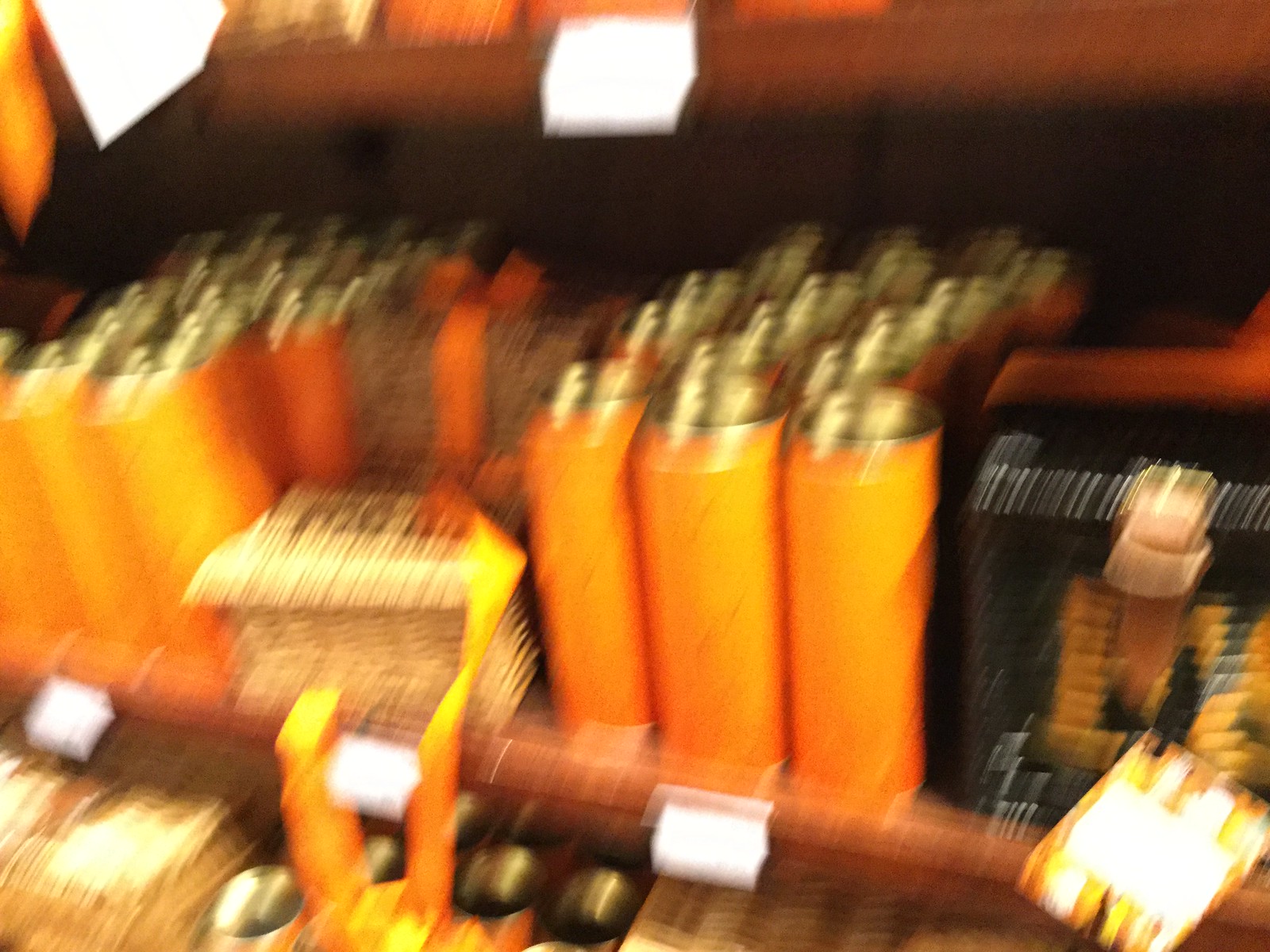This photograph, taken inside a store, captures a blurry scene dominated by a mid-level shelf. The shelf houses various items, although their exact details are obscured due to the image blur. Predominantly, there are tall, orange-colored bottles or cans with gold tops, organized into at least two distinct groups. These groups extend back three to four items deep. 

Between these groups of orange containers, a small rectangular wicker basket is visible, with some letters or numbers that are unreadable. Another similar wicker basket is placed to the right of the orange cans, displaying what appears to be a yellow ribbon and possibly containing items such as pads of butter or pieces of chocolate. Additionally, a black box with yellow markings lies next to these wicker baskets. White price tags are positioned beneath the various items on the shelf, indicating their placement for sale. The photo is overall blurry, suggesting that the camera was in motion when the shot was captured.